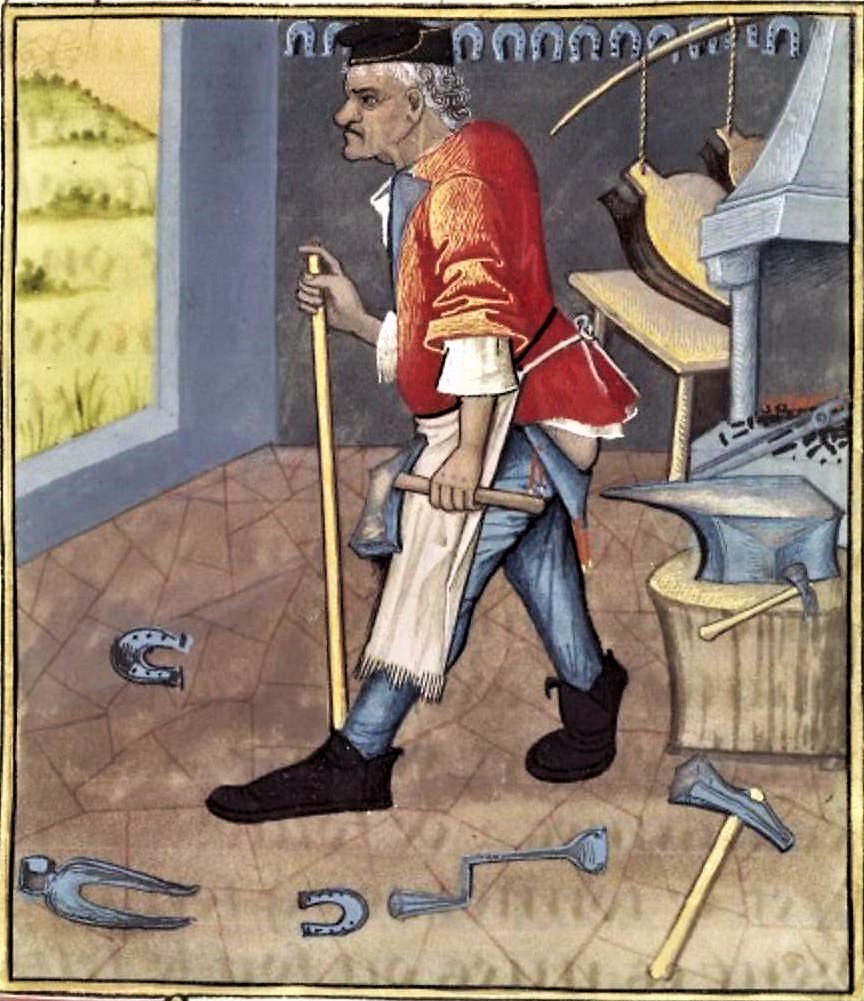This image is an illustrated scene depicting a blacksmith from what appears to be colonial times. The man is centrally placed within the picture, exuding a somewhat humorous tone due to his sagging blue pants that reveal a bit of his behind. He is wearing a red colonial jacket over a white shirt, with a white apron tied around his waist, and oversized black shoes. His head is adorned with a black beret, and his facial expression appears grumpy, framed by white hair.

In his right hand, he holds a walking stick that extends from his mid-chest to the floor, and in his left hand, he clutches an axe. Surrounding him are various tools indicative of his trade: to his right lies a horseshoe, and to his left are ironworking tools along with another axe. A metal fireplace with tongs protruding from it, usually for heating and bending metal, can be seen behind the log-mounted anvil.

The setting includes a gray wall adorned with horseshoes at the top, and an old-fashioned tan hand pump fan rests on a white pine table. Through a window on the right side of the image, a grassy hill is visible, adding depth to the background. Additionally, the illustration seems to have an uneven border, as if it was cut out from an old newspaper comic strip, suggesting it might be a snippet from an antique publication.